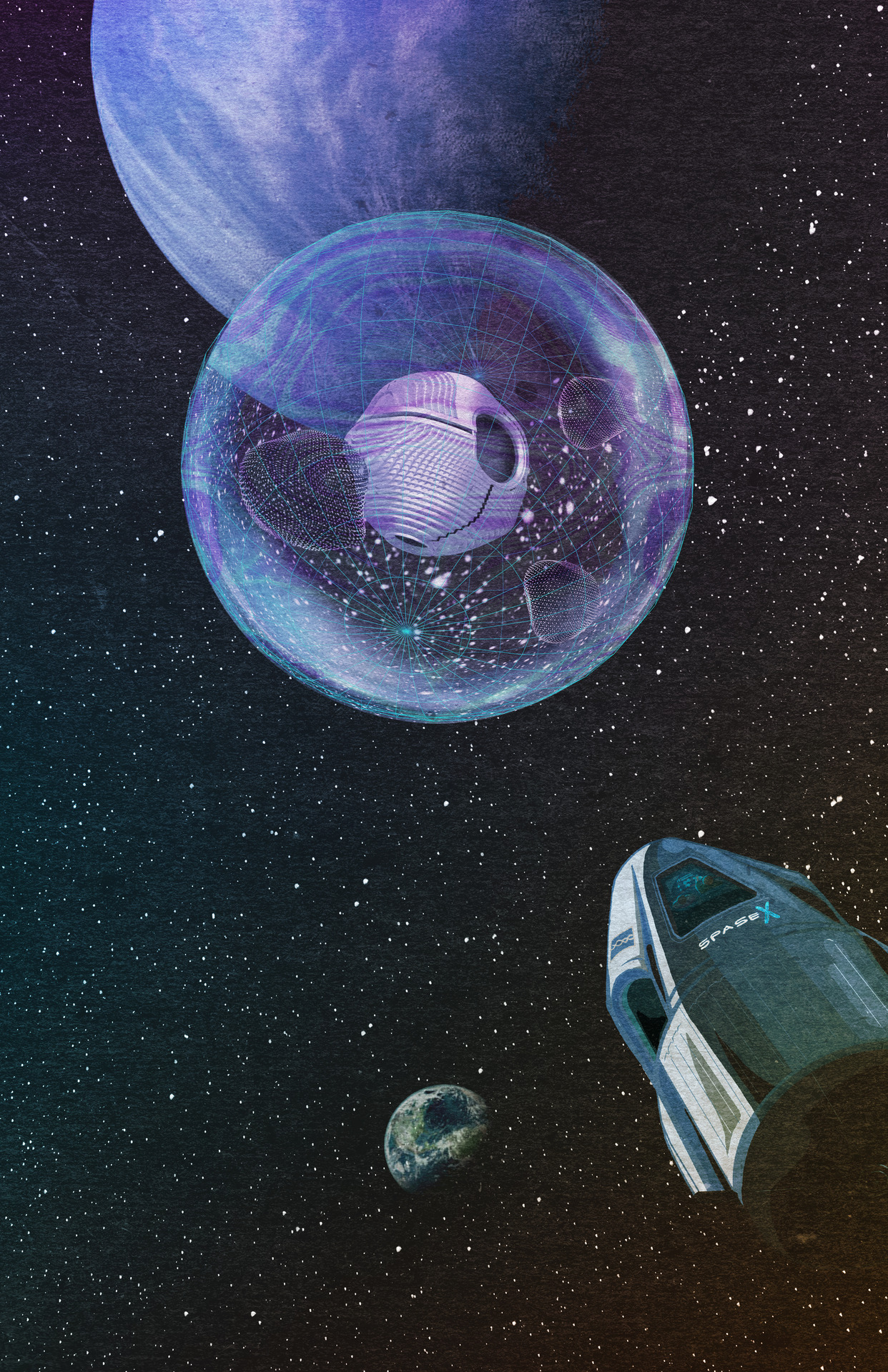This high-quality digital science fiction artwork depicts a captivating outer space scene. The black background is speckled with thousands of tiny white stars, creating a vast and mysterious cosmos. At the bottom center of the composition, Earth is portrayed with its characteristic blue, green, and white swirls. To the right of Earth, a SpaceX Dragon crew module is prominently featured, clearly marked with the "SpaceX" logo—the "X" standing out in light blue.

At the top-central area of the artwork, a massive blue gas giant with swirling white clouds looms, adding depth and intrigue to the scene. Between this gas giant and the SpaceX craft, there is a mesmerizing, translucent bubble-like structure with a shimmering oil-and-water effect and a gridded surface. Inside this enigmatic bubble are four spherical objects: a central white sphere with two large black openings and smaller black dots, surrounded by three other spheres that have a pink outline. The SpaceX craft appears to be heading towards this mysterious bubble, potentially investigating the alien artifact within. The entire composition beautifully balances elements of realism with the imaginative essence of science fiction.